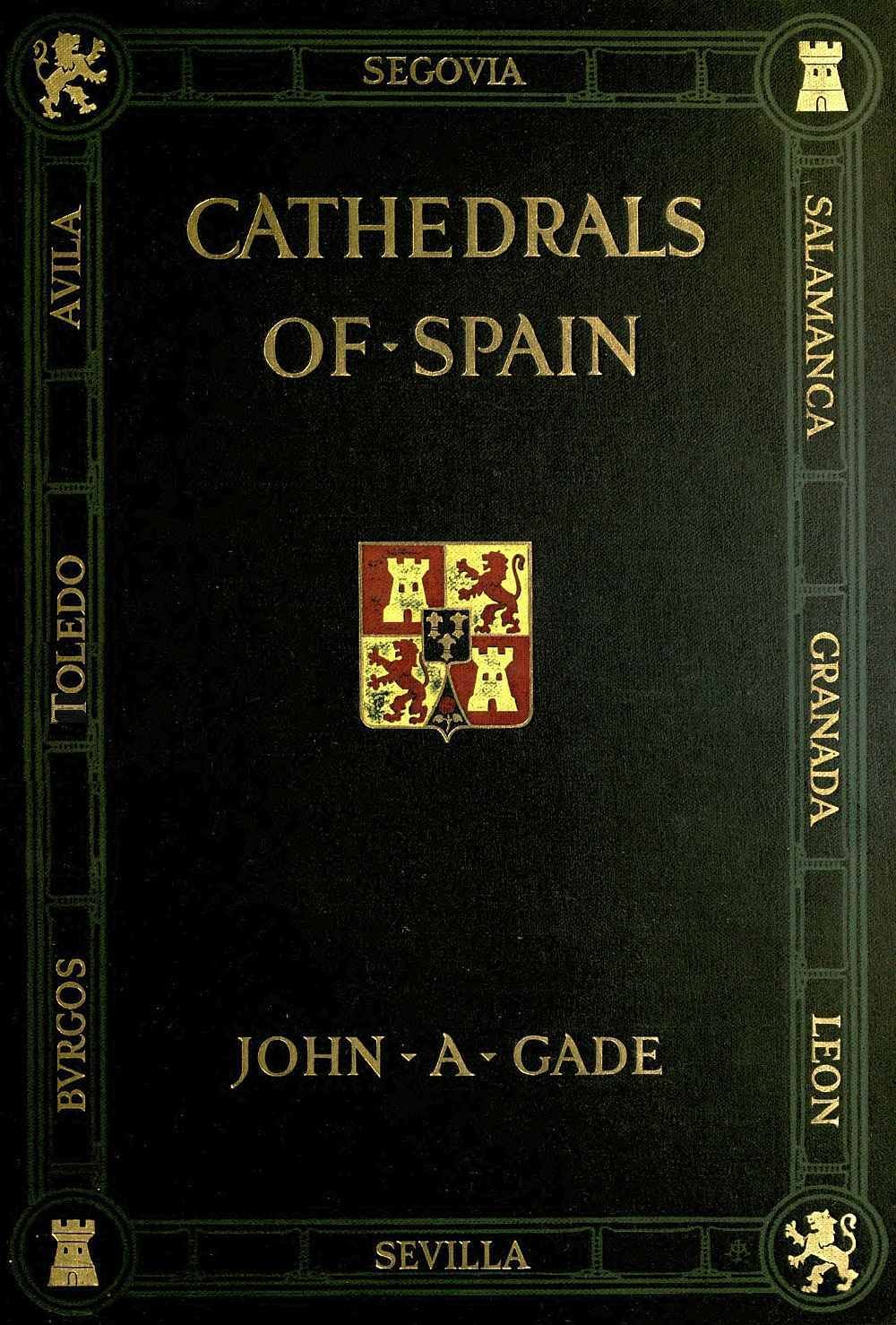The cover of the book "Cathedrals of Spain" is depicted with an intricate design. The background is a dark green color, featuring the book’s title, "Cathedrals of Spain," in gold text at both the top and bottom. The author, John A. Gade, is mentioned at the bottom in matching gold text. At the center of the cover, a detailed coat of arms is presented. This coat of arms is divided into four sections: the top right and bottom left quadrants display a red lion against a white background, while the top left and bottom right quadrants feature a white castle against a red background. Additionally, a blue shield occupies the central position of the coat of arms, complemented by a red rose below it. Surrounding the central image, the book cover has a border listing the names of various Spanish cities, including Segovia, Salamanca, Granada, Leon, Sevilla, Figueros, Toledo, and Avila, with circular embellishments at the corners. The overall layout of the book cover is rectangular and set in a portrait orientation.